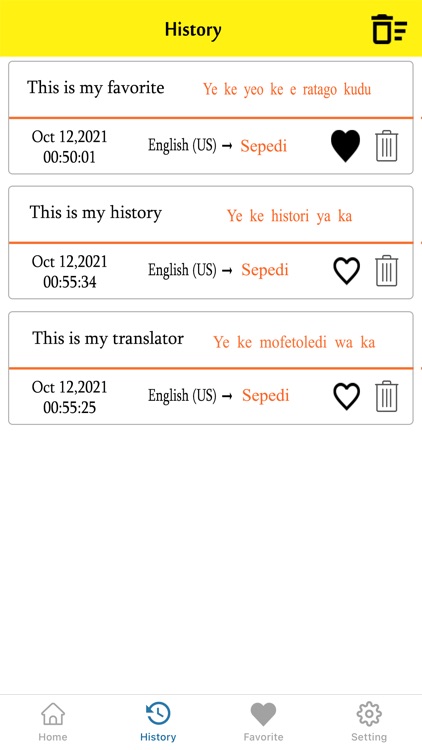**Detailed Caption for the Screenshot of a Mobile App's History Page:**

The image is a screenshot of the history page within a mobile app. The interface is user-friendly and visually structured for easy navigation.

At the top of the screen, there is a yellow header with the word "History" prominently centered in black font. To the right of this header are two icons: a trash can icon for deleting entries and a menu icon for additional options.

The main body of the page is white, providing a clean and clear background for the listed items. At the very top of the history entries, there is a bar that reads "This is my favorite" with a segment of red text displayed to the right in a different language.

Below this, the first entry is highlighted with noticeable details:
- On the left, the date "October 12th, 2021" is shown, followed by the exact time below it.
- In the center, the text "English (US) to Sepedi" is displayed, with "Sepedi" highlighted in red.
- On the right, there is a heart icon filled in black to indicate it has been selected (favorited), along with a trash can icon at the far right for deletion.

The subsequent entry on the list includes similar details:
- The entry reads "This is my history," with another segment of red text on the right in a different language.
- Again, the date and time "October 12th, 2021" are displayed on the left.
- The middle text states "English to Sepedi," with "Sepedi" highlighted in red.
- On the right side of this entry, there is an unselected heart icon followed by an unselected trash can icon.

At the bottom of the screenshot, there is a statement that reads "This is my translator," signifying the purpose of the app.

Overall, the screenshot effectively captures the functional and aesthetic elements of the mobile app's history page, detailing the user's activity and preferences within the app.